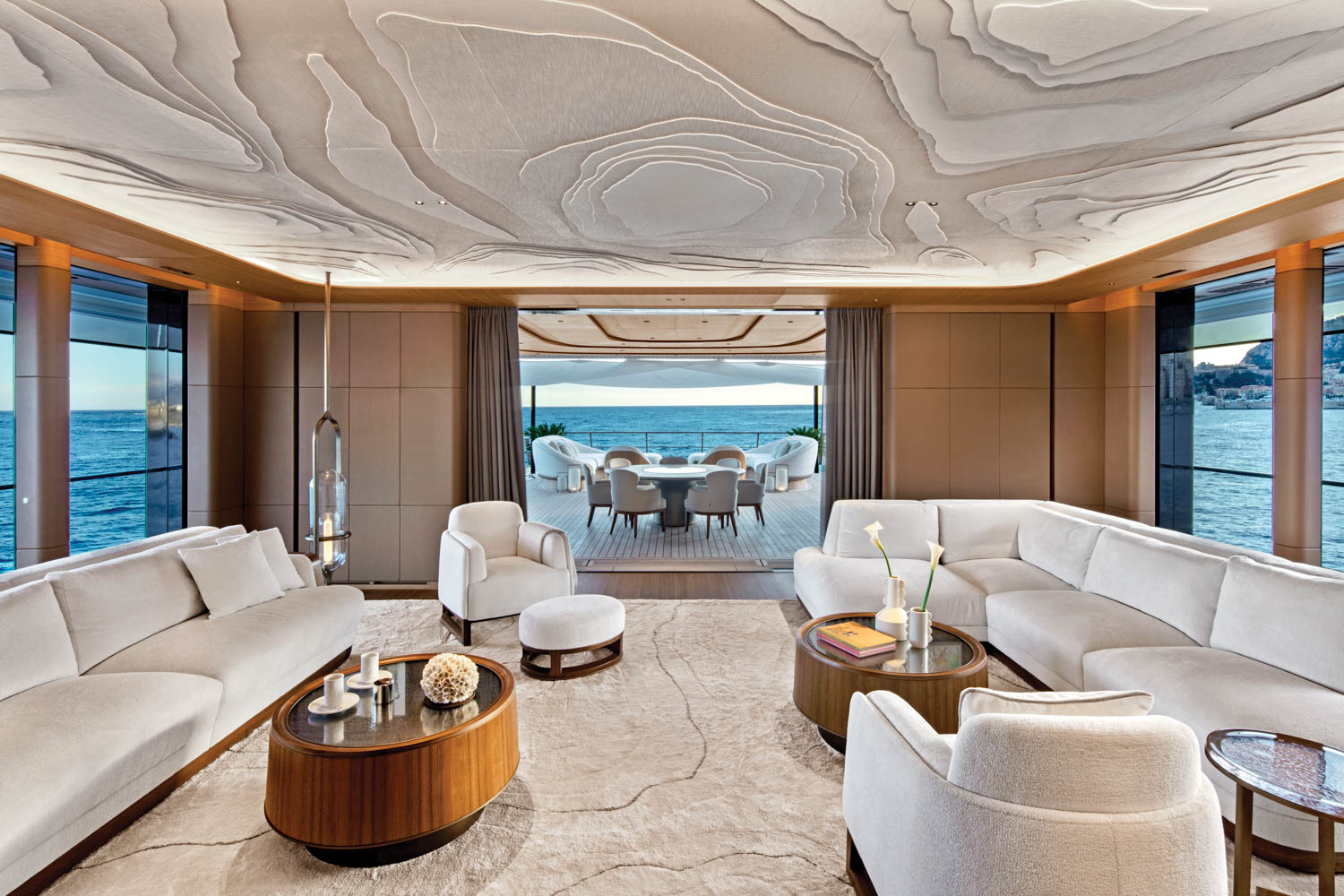This photograph captures the luxurious interior of a yacht, bathed in natural light from the large windows framing the view of the surrounding ocean. The room features plush white upholstered furniture, including an L-shaped sectional sofa and armchairs with ottomans, arranged on a lavish beige carpet laid over rich brown hardwood floors. Multiple round and oval wooden tables, some with glass tops, hold various decorative items such as coffee table books, white vases with irises, and artistic ornaments. A standout feature of the room is its intricate, topographically textured white ceiling. The space is framed by beige curtains and furnished with pendant lights hanging from the ceiling.

Toward the back of the room, an opening leads to a deck through a doorway draped with curtains. The deck itself is equipped with dark-colored rails and features more white upholstered furniture, including two deck chairs and a round outdoor dining table surrounded by chairs, all positioned to take advantage of the stunning ocean views. The overall ambiance is one of opulence and comfort, befitting a high-end yacht.